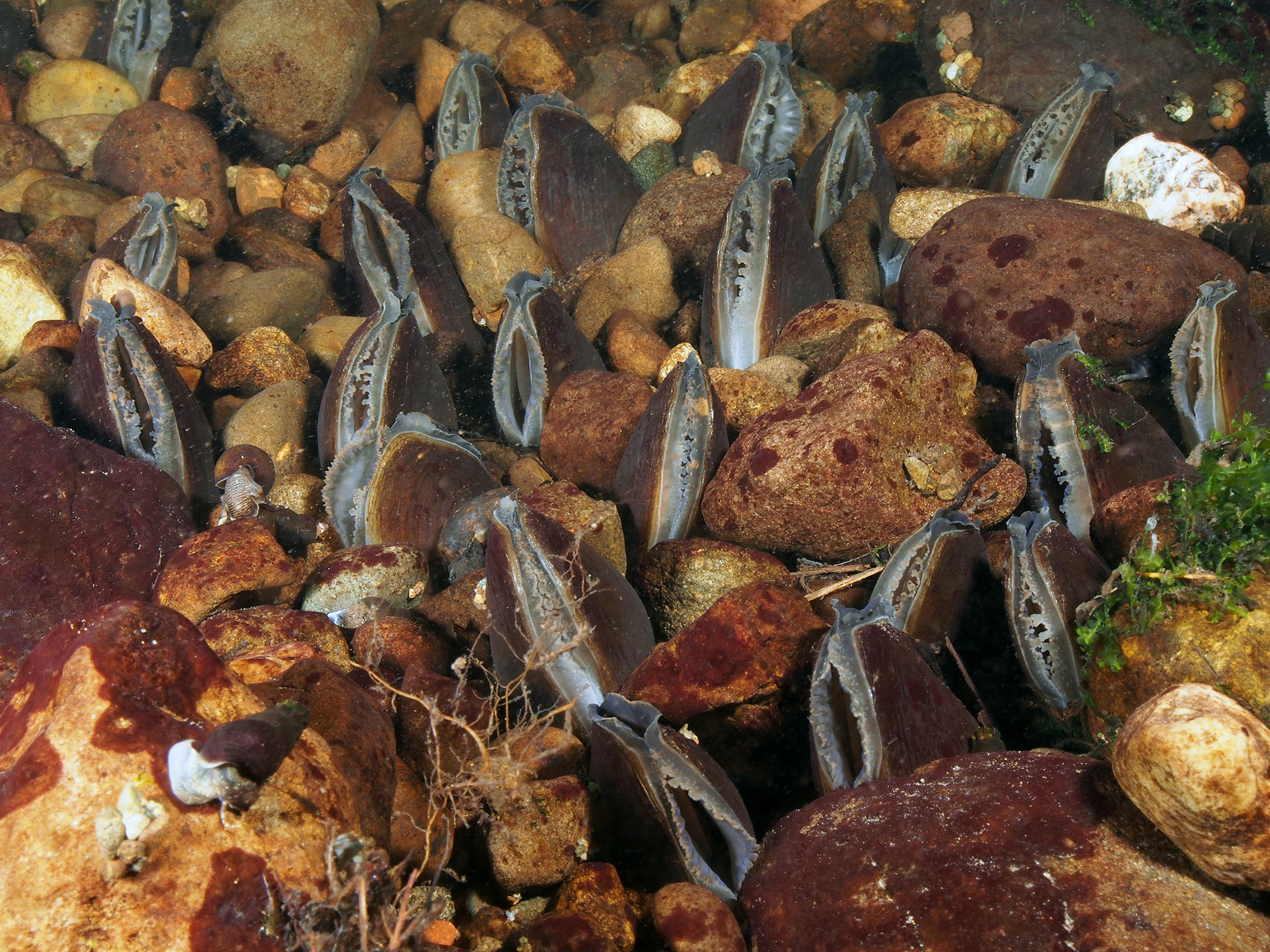The underwater photo depicts a vibrant and detailed scene of the ocean floor, blanketed in rocks of varying shades of brown. Among the rocks, over a dozen brown clams or mussels are nestled, their sides slightly open, revealing bluish-gray insides. These bivalves appear to be feeding, possibly filtering water for plankton or small fish. Scattered across the image are small green plants and roots, with some barnacles attached to the rocks. On the front left portion of the scene, a snail is visible, clinging to a rock. The overall image is well-lit, showcasing the intricate details of the underwater ecosystem.